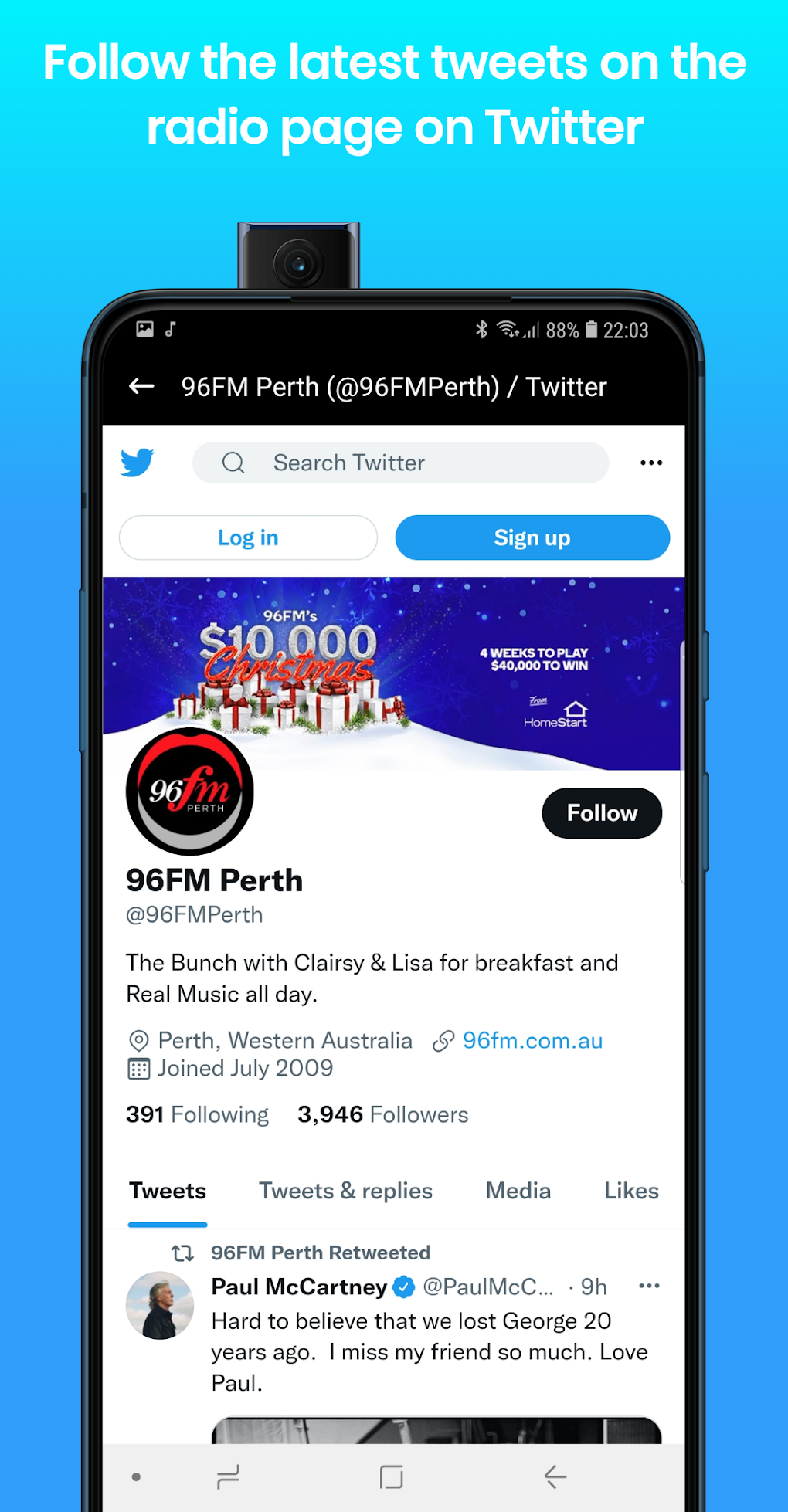The advertisement features a visually appealing background gradient transitioning from aqua at the top to a lighter blue towards the bottom. At the top of the image, large white text reads, "Follow the latest tweets on the radio page on Twitter." Below this text, there is an image of a cell phone displaying the 96FM Perth Twitter page. The account handle, "@96FMPerth," is prominently shown. The screen of the phone displays a tweet from Paul McCartney, dated to commemorate the 20th anniversary of George Harrison's passing. The tweet reads, "Hard to believe that we lost George 20 years ago. I miss my friend so much. Love, Paul." The Twitter interface also shows options to log in or sign up, further encouraging viewers to engage with 96FM Perth on Twitter.